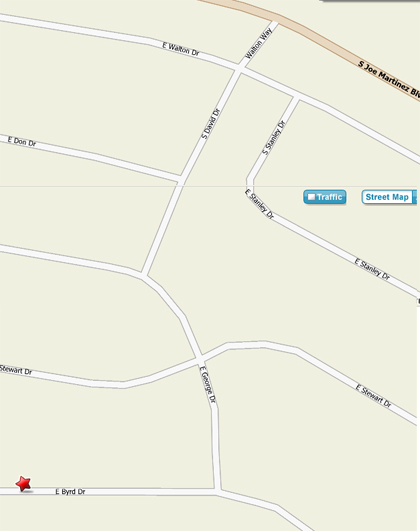This detailed vertical image features a street-level view of a map, reminiscent of a Google Maps interface. The map showcases various roads, primarily depicted in white, with a significant road at the top right corner highlighted in a light brown hue. Street names are meticulously labeled in small black letters. A prominent red star marks a specific location on a street in the bottom left corner. Towards the top right, a mouse pointer arrow hovers over an empty area on the map. Centrally positioned to the right, a blue rectangle with the word "Traffic" in white is prominently displayed. Adjacent to it, within a white box outlined in blue, the words "Street Map" appear in blue font. The overall background of the map is a light tan color, providing a clear and aesthetically pleasing view.